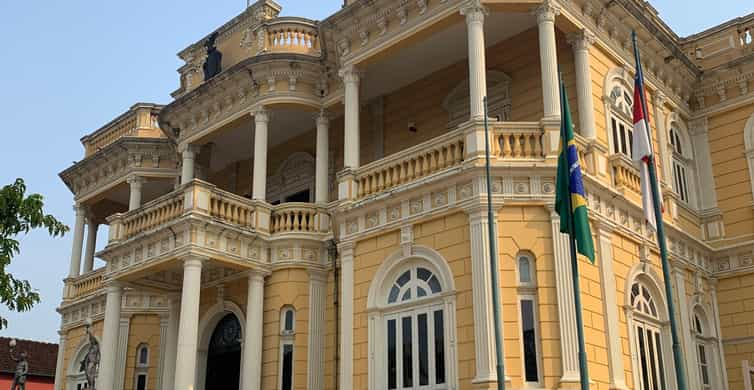The image captures a grand and elegant yellow architectural structure, potentially a historical building or mansion that exudes a majestic and stately presence. Painted in bright yellow with contrasting white trimmings, the building features multiple large windows with arched tops and intricate detailing, adding to its sophisticated appearance. Prominent balconies boasting ornate railings highlight the second story, where a spacious patio invites one to enjoy views of the surroundings. 

At the forefront, a set of grand stairs leads up to an impressive main entrance, adorned with imposing columns and a large white archway, enhancing the building's grandeur. Standing tall on the right side are three flagpoles; the central pole proudly flies the Brazilian flag, characterized by its green, yellow, and blue colors, while the poles flanking it showcase a red and white flag and an empty pole. The scene is set against a backdrop of a clear, light blue sky with some visible tree branches on the left, framing the image beautifully. The overall impression suggests that this might be an important or historical government building, potentially in Brazil, given the prominence of the Brazilian flag.